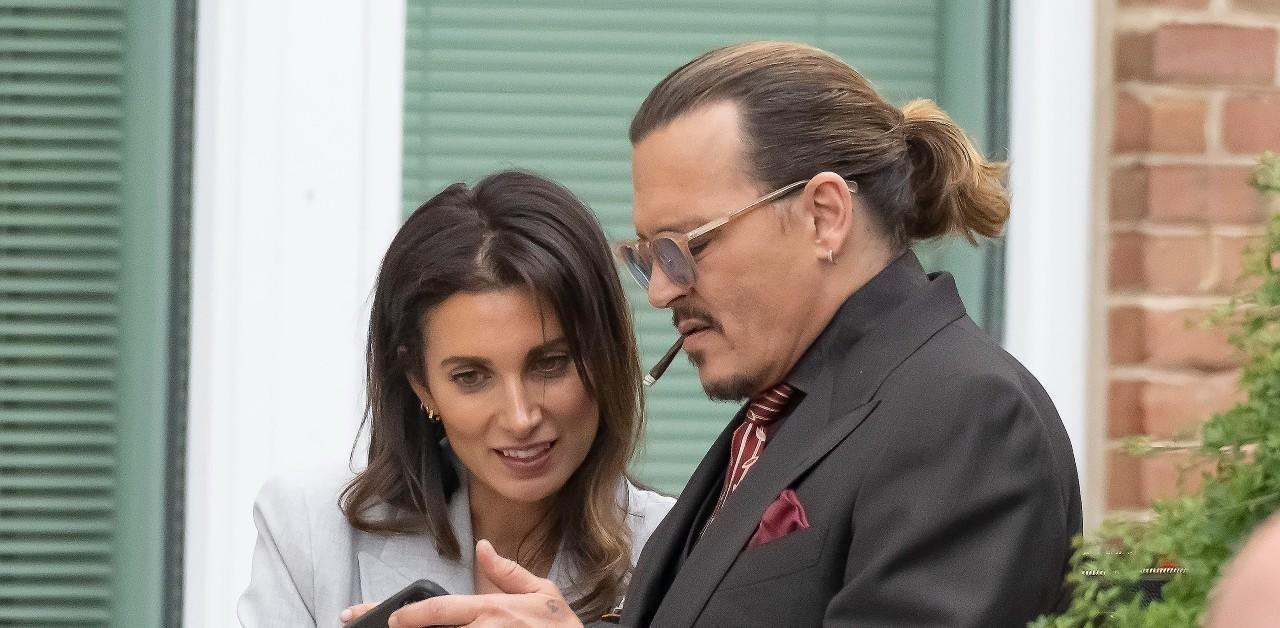In this vibrant daytime outdoor photograph, Johnny Depp stands at the center in front of a brick building, accompanied by a stylish woman with long brown hair. Both are fixated on a cell phone that Depp holds in his hands. Depp is impeccably dressed in a dark, possibly gray or black suit, complemented by a maroon or purple pocket square and matching tie. His hair is slicked back into a ponytail, and his left ear sports a hoop earring. He wears sunglasses and has a small cigarillo perched on his lips, accentuating his mustache and chin beard. The woman beside him, elegantly attired in a white suit jacket and blouse, gazes at the phone with a slight smile. The background features white blinds in the windows and green shutters, with a bush partially visible in the lower right corner, adding a touch of greenery to the scene.